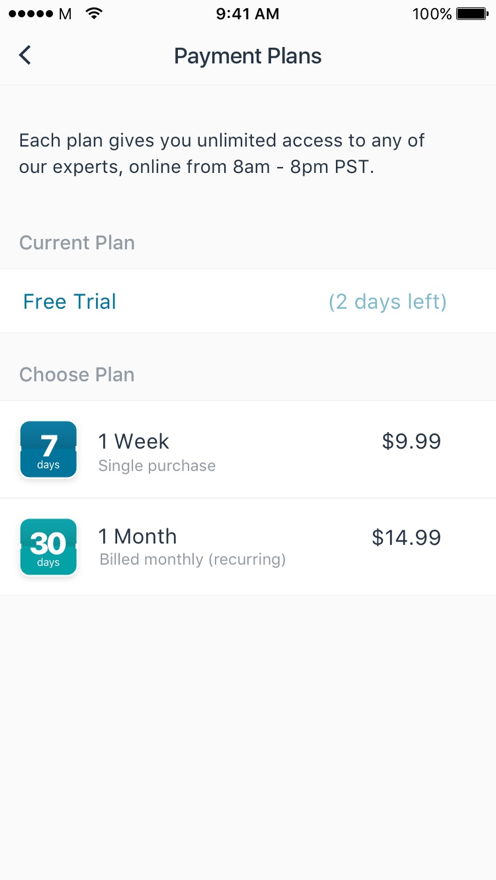A detailed smartphone screenshot is displayed against a white background. At the very top center, the time is shown as "9:41 AM" in black font. In the upper right corner, there is a battery icon indicating a full charge at 100%, while in the upper left corner, five black dots signify a strong wireless connection, next to a capital letter "M" and a Wi-Fi icon.

In the center, the title "Payment Plans" is prominently displayed. To the left of this title, an arrow points to the left, suggesting a navigation option. Below, a gray font message reads, "Each plan gives you unlimited access to any of our experts online from 8 AM to 8 PM PST."

On the left side, the text "Current Plan" in gray font is followed by "Free Trial" in blue font. To the right of this, within parentheses, it states, "2 days left." Below this section, "Choose Plan" is written in gray font.

Two plan options are listed beneath:
1. "One Week Single Purchase" is accompanied by a blue square containing a white number "7," with the price on the right listed as $9.99.
2. "One Month" marked as "Billed Monthly Recurring," is highlighted with an aquamarine green square housing a white number "30," with the price listed as $14.99.